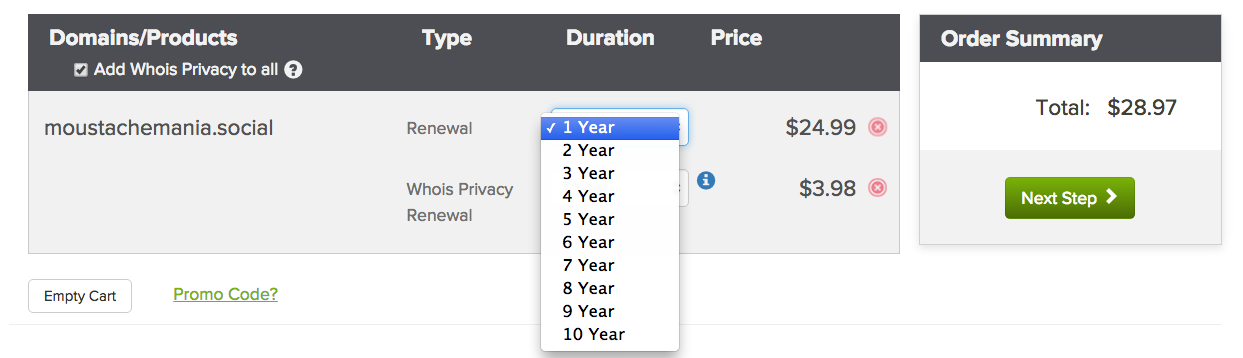This image captures a desktop screenshot showcasing a software checkout screen for purchasing and renewing domain services. Dominating the top left of the screen, a dark gray rectangle features the white, bolded text "domain/products." To the right, columns labeled "Type," "Duration," and "Price" are visible, indicating the specifics of items in the cart. A small checked checkbox with the text "Add WHOIS privacy to all" is present, accompanied by a gray question mark in a white circle, suggesting additional information is available.

The displayed domain is "moustachemania.social," with the type set to "Renewal." The duration option ranges from one to ten years, with one year currently selected, priced at $24.99. There's a red 'X' icon allowing removal of this item from the cart. Below, an option for "WHOIS Privacy Renewal" is available, likely offering the same duration options though not fully visible. It costs $3.98 and includes a blue circle with a white 'i' for more information, along with a removal option.

Further down, options to "Empty Cart" or enter a "Promo Code" appear in green text. On the right side, a dark gray rectangle with white text reads "Order Summary," detailing a total of $28.97 USD. Below, a green rectangle with white text "Next Step" and an arrow highlights the action button.

This checkout screen is tailored for purchasing rights to the domain "moustachemania.social" and WHOIS privacy protection, summarizing the pertinent details for the transaction.